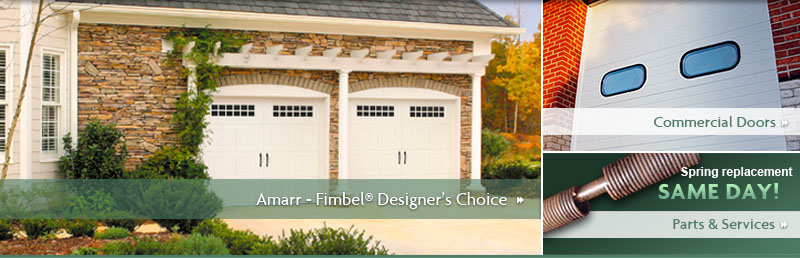This is a detailed screenshot showcasing a mock-up or an active webpage for a garage door repair and installation service. The left two-thirds of the image feature a tightly cropped view of a house with an elegant stone facade, highlighting two side-by-side, well-crafted garage doors. To the right of this image, text reads "Amar Fimble, Designer's Choice" followed by two smaller images stacked vertically.

The top image displays a brick garage with a unique garage door, featuring two portal windows. The caption beneath this image reads "Commercial Doors." Below this is another image of a large spring set against a green background with text reading "Spring Replacement Same Day." Additionally, there's a button labeled "Parts and Services."

Each text section includes double arrows pointing to the right, indicating hyperlinks to further details or separate sections. Notably absent from the webpage are distinct branding elements or logos, making it unclear if this screenshot is from an actual website or just a design mock-up. Regardless, it effectively represents a company involved in the repair and installation of garage doors.